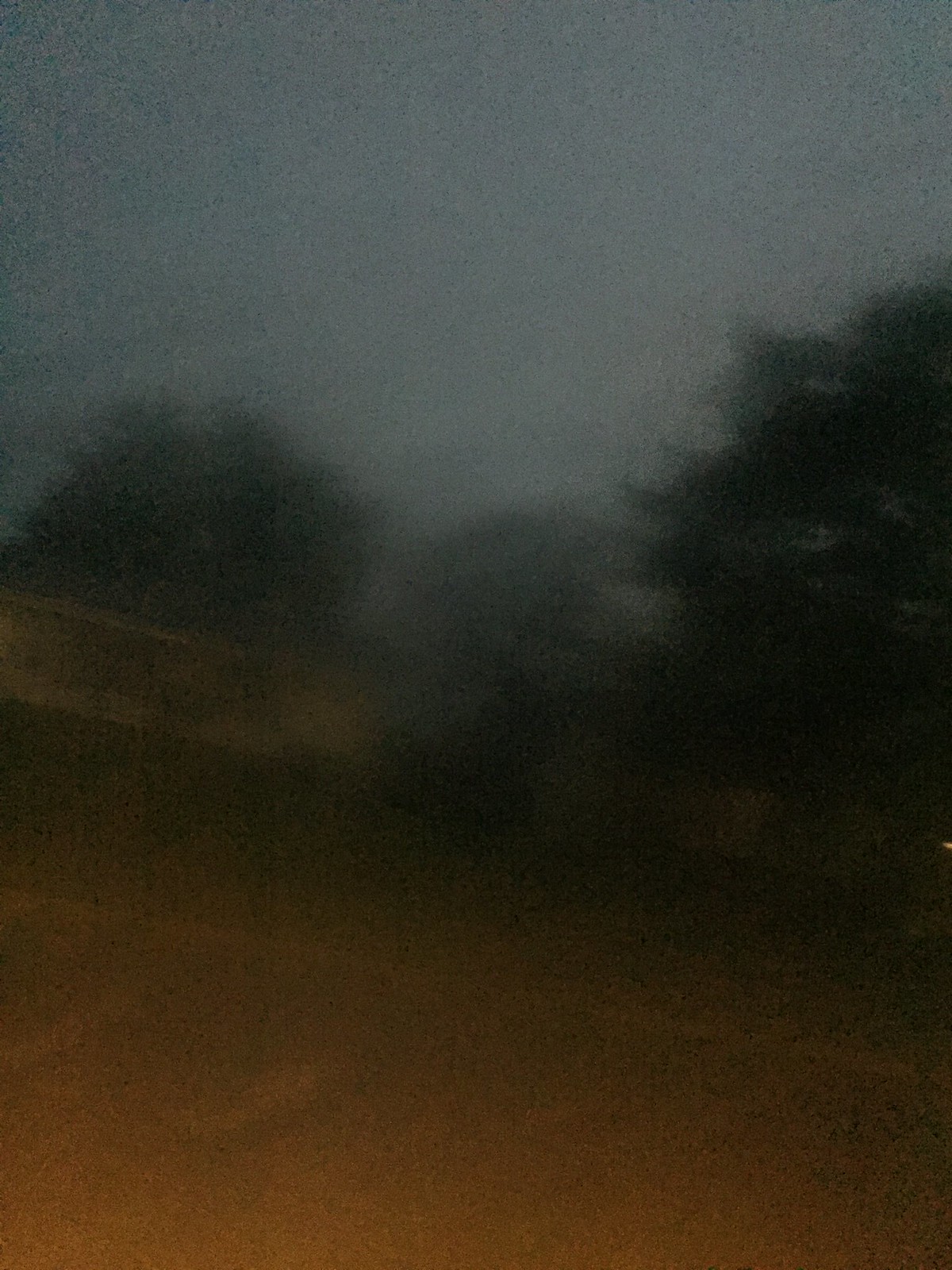This is a very blurry photograph taken at night, depicting an indeterminate scene with a clear sky devoid of the moon, stars, or twilight. The image features the silhouettes of various trees, displaying a gradient of green hues. On the right-hand side, the trees appear the darkest in color, while the center trees are a lighter shade, and the left-hand side presents a mid-range green. In the foreground, there seems to be a dirt road or dirt parking lot suggested by the presence of brown tones. A distinct line separates this foreground from the background trees.

In the middle of the image, there is an indistinct, long, rectangular object running horizontally across the trees. This object could potentially be a guardrail, a series of boards, or a sign that lacks clarity. There is a noticeable break in this object, followed by another rectangular object, positioned at about waist height.